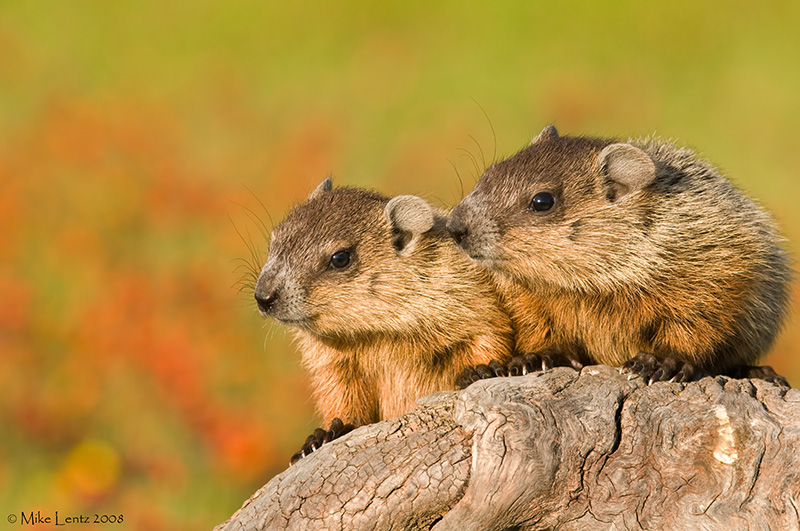In this vibrant 2008 photograph by Mike Lentz, two prairie dogs—or possibly other small rodents—are captured in a natural setting, perched atop a gnarled piece of wood. Their curious eyes and dark brown noses peek out as they sit side by side, both gazing towards the left. The distinct fur coloring is notable: their heads are a darker brown, transitioning to a lighter golden brown down their necks and bellies, with their backs appearing more grayish. The wood beneath them is richly textured, full of knots and crevices. The backdrop, though blurred, adds a splash of color with greens, reds, and oranges, likely representing a field of grass and flowers. The overall composition is bathed in sunlight, enhancing the earthy tones of the scene. In the lower left corner, the image is signed "Mike Lentz 2008" in black font, asserting the photographer's credit.